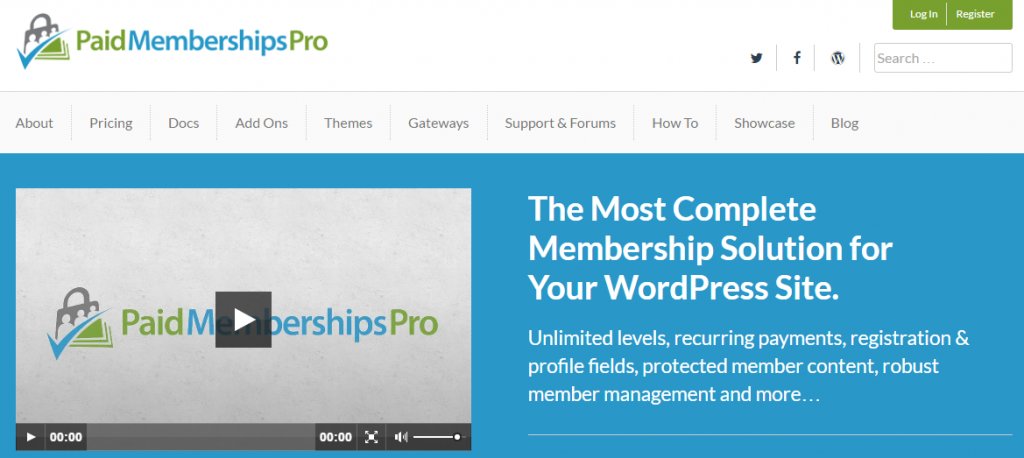In the image, the top right corner displays the text "Paid Memberships Pro," with "Paid" and "Pro" in green and "Memberships" in blue, all written as a single phrase without spaces. To the left of this text is a logo featuring a blue check mark and a suitcase with three person silhouettes inside. On the far right, there are green boxes containing "Login" and "Register" in white text.

Below this top section, to the left, are icons for social media: a bird icon for Twitter, the letter "F" for Facebook, and a "W" icon. Beneath these icons are various categories presented in separate boxes and separated by lines. The categories, from left to right, include: About, Pricing, Docs, Add-ons, Themes, Gateway, Support, Forums, How-to, Showcase, and Blog.

Underneath the text "Paid Memberships Pro" and the category boxes, there is a video player with a play button in the center. To the right of the video, text describes the service as "the most complete membership solution for your WordPress site," highlighting features such as tiered membership levels, recurring payments, registration and profile fields, protected member content, robust member management, and more.